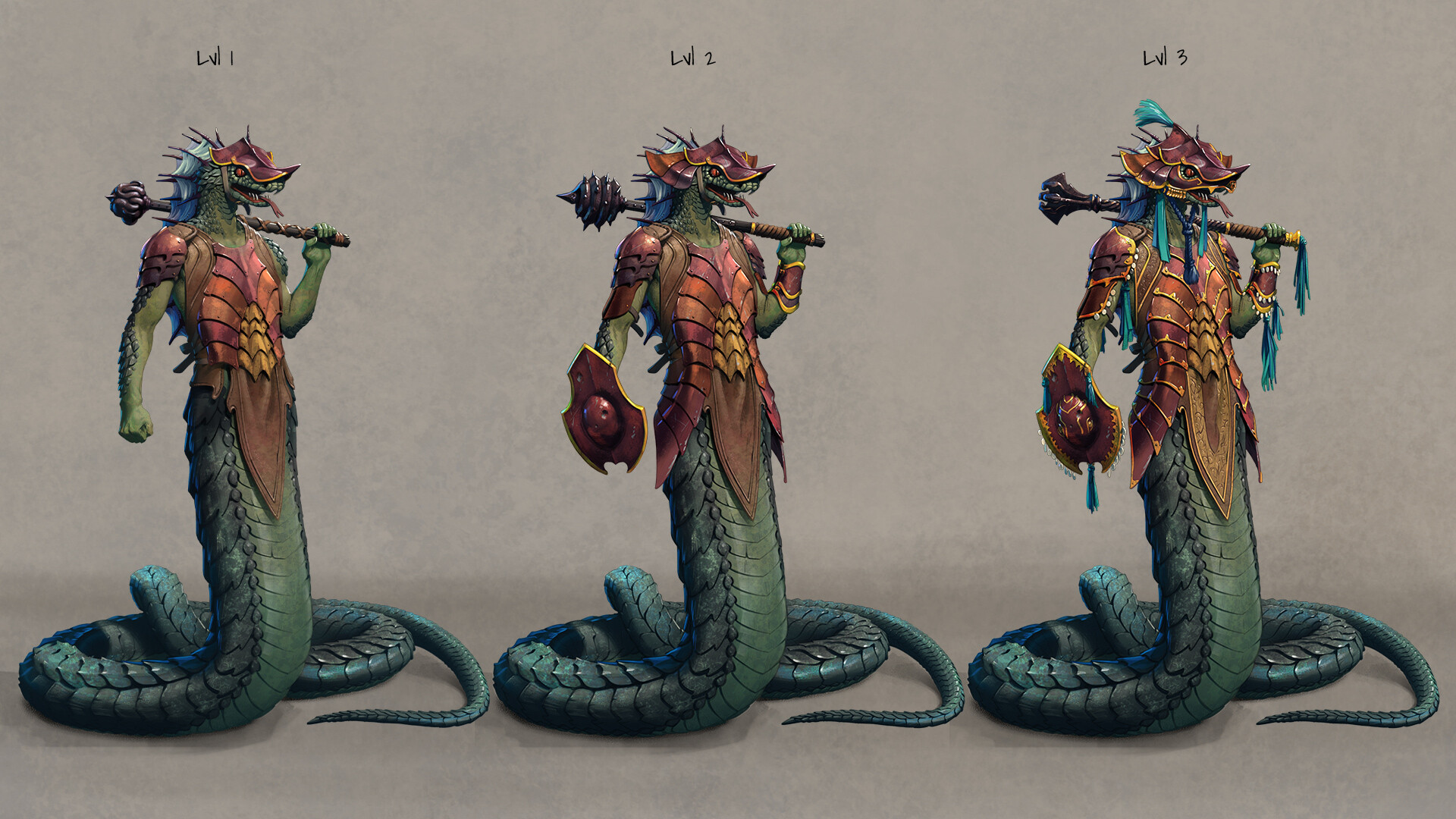This image features a triptych display of three human-like lizard creatures, seemingly from a futuristic or fantastical video game. Each creature is adorned with armor made of scales, and has blue fins extending from behind their heads down to their backs. They all share a similar green coloration and possess long, thick tails instead of legs. In their left hands, they hold weapons defined by circular designs at the edges. The creatures are labeled LVL 1, LVL 2, and LVL 3 from left to right, indicating a progression in their form and equipment. The LVL 1 creature is the most basic, while the LVL 2 creature features additional frills on its head and a more elaborate shield and scepter. The LVL 3 creature is the most advanced, with the most sophisticated armor and weaponry, including a pendent-like addition to its shield. The presentation appears CGI-generated, emphasizing the characters' roles within a video game or animated storyline.